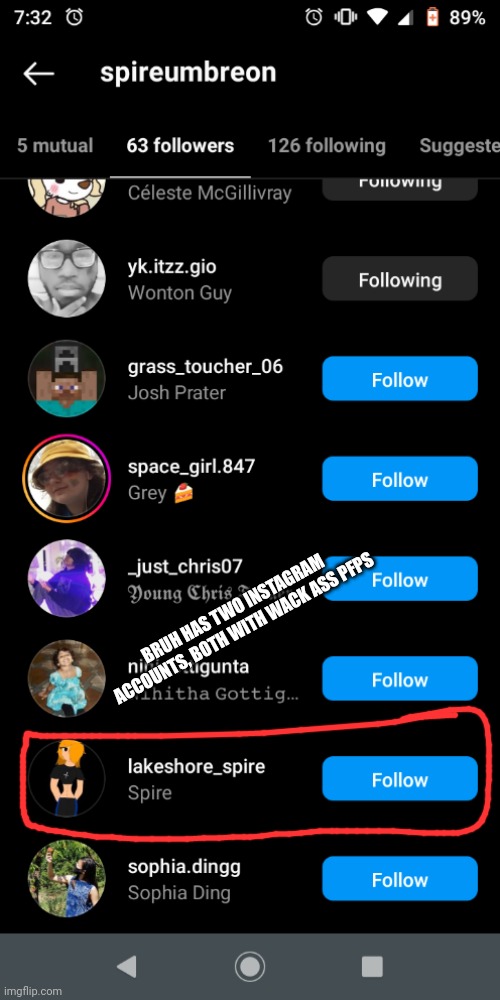Captured on a cell phone, the image depicts what appears to be a social media page with a highlighted user profile. The top left corner indicates the time as 7:32 with an accompanying clock icon, while the top right corner displays icons for Wi-Fi signal, battery life at 89%, and another clock. The user's handle "Spireumbrion" (S-P-I-R-E-U-M-B-R-E-O-N) is shown next to a white left arrow. Directly below this are statistics and options, including "5 mutual," "63 followers," and "126 following," alongside a "suggested" section.

In the suggested section, several profiles are listed with small avatars:
- Celeste McGillivay (following)
- YK.ITZZ.GIO (following)
- Grass_toucher-06 (Josh Prater) with a blue "Follow" button
- Space_girl.847 (gray, with a cake emoji) with a blue "Follow" button
- \_just\_Chris07 with a blue "Follow" button

At the center of the image, in white text, it reads: “bruh has two Instagram accounts, both with whack ass PFPS.” Below this, the username "Lakeshore_Spire" is displayed with a blue "Follow" button, prominently circled in red to draw attention.